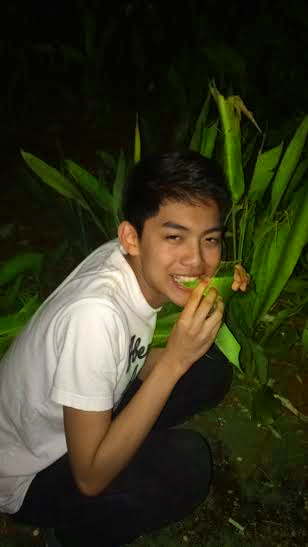The photograph captures a young Asian boy, likely around 15 or 16 years old, kneeling in a garden area outdoors at night. He has short black hair and dark eyebrows, and his thin arms complement his lean build. He is smiling widely, showcasing his teeth, as he gazes directly at the camera. He wears a white short-sleeved t-shirt with black writing, partially readable as "ABE," hinting at an Abercrombie & Fitch design, and pairs it with black pants.

The boy is in a playful posture, squatting and holding a long, bright green leaf with both hands near his mouth, pretending to bite it. The surrounding vegetation features a medium-sized plant with tall, vibrant green leaves contrasting against the dark brown ground. The photograph’s background is pitch black, indicating it was taken at night with a flash, further emphasizing the boy and the lush greenery around him.